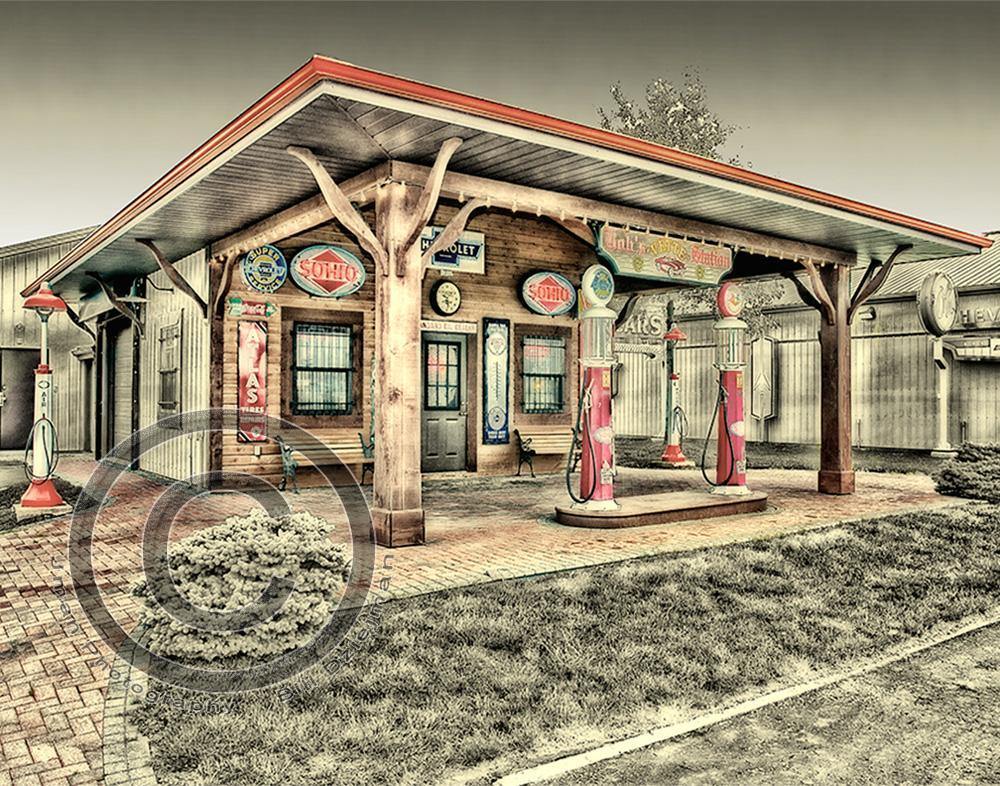This detailed digital artwork depicts an old-fashioned gas station reminiscent of the 1930s and 40s in the USA, rendered predominantly in various shades of gray. The scene is set against a gray sky, enhancing the vintage ambiance. The primary focus is a wooden building with metal sides, positioned diagonally in the image, featuring a prominent overhang supported by thick wooden beams that creates an arcade-like area. This overhang shelters two pale red gas pumps with clear glass tops displaying indistinct gas brand names.

The front facade of the gas station showcases multiple windows and a central door, adorned above with several indistinguishable old signs, including faint references to "Chevrolet" and "Soho." The surrounding environment, including the grass and a bush on the right, is also rendered in gray tones, contributing to the nostalgic feel. A walkway runs beneath the overhang, curving from the front of the building to the left side and extending towards the bottom left of the image. In the background, a gray tree and a long metal fence stretch behind the building, while a large gray circle with a "C" in the middle is visible on the left side, further enhancing the vintage motif of the scene.